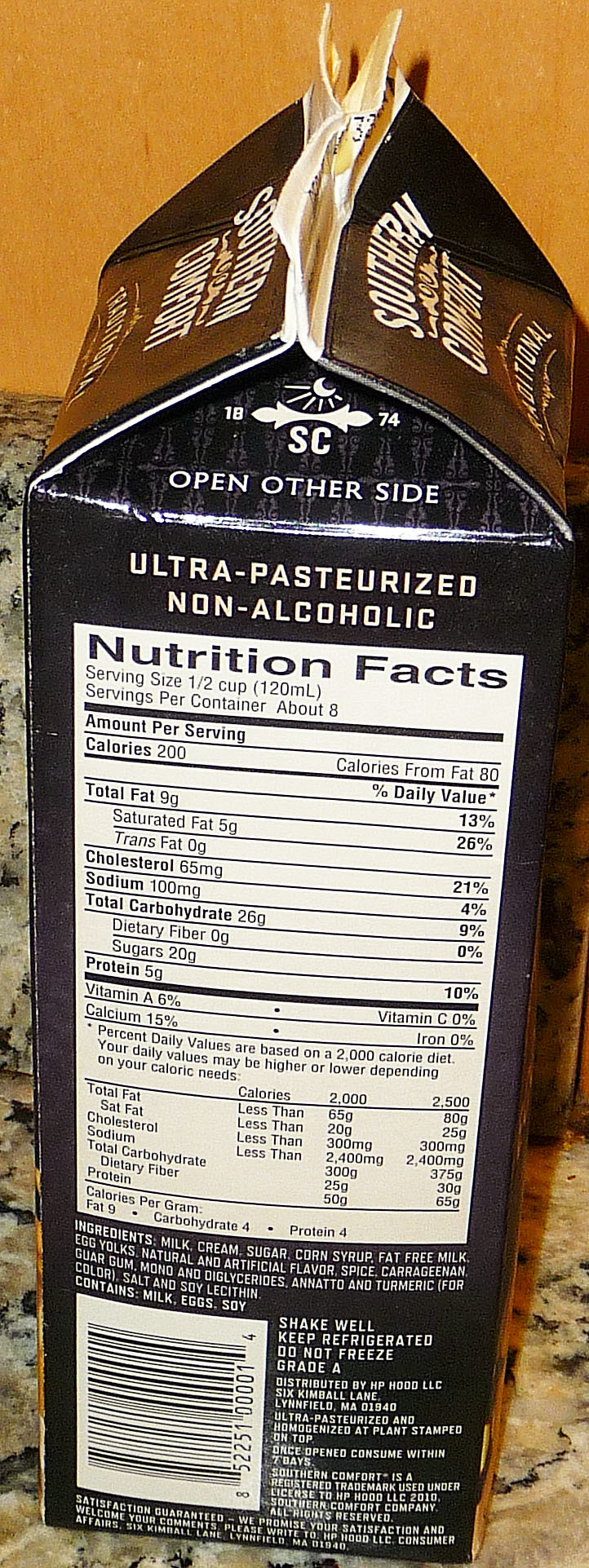This color photograph captures a detailed side view of a one-quart milk carton-style container. The carton predominantly features a brown front and back, with the visible side panel distinguished by a black background. The front label appears to bear the name "Southern Comfort," suggesting a brand association, though this particular product is non-alcoholic, as indicated by the text "ultra-pasteurized, non-alcoholic" printed clearly on the side.

The side panel prominently displays a white Nutrition Facts label. A half-cup serving of the beverage contains 200 calories. While some of the nutritional values are difficult to read, it faintly shows that the product contains 20 grams of sugar and 9 grams of fat. Toward the bottom of the panel, a barcode and a list of ingredients are visible in white text against the black background, but they are too small to be legible. The overall composition provides a clear, albeit incomplete, view of the nutritional and branding aspects of the carton.